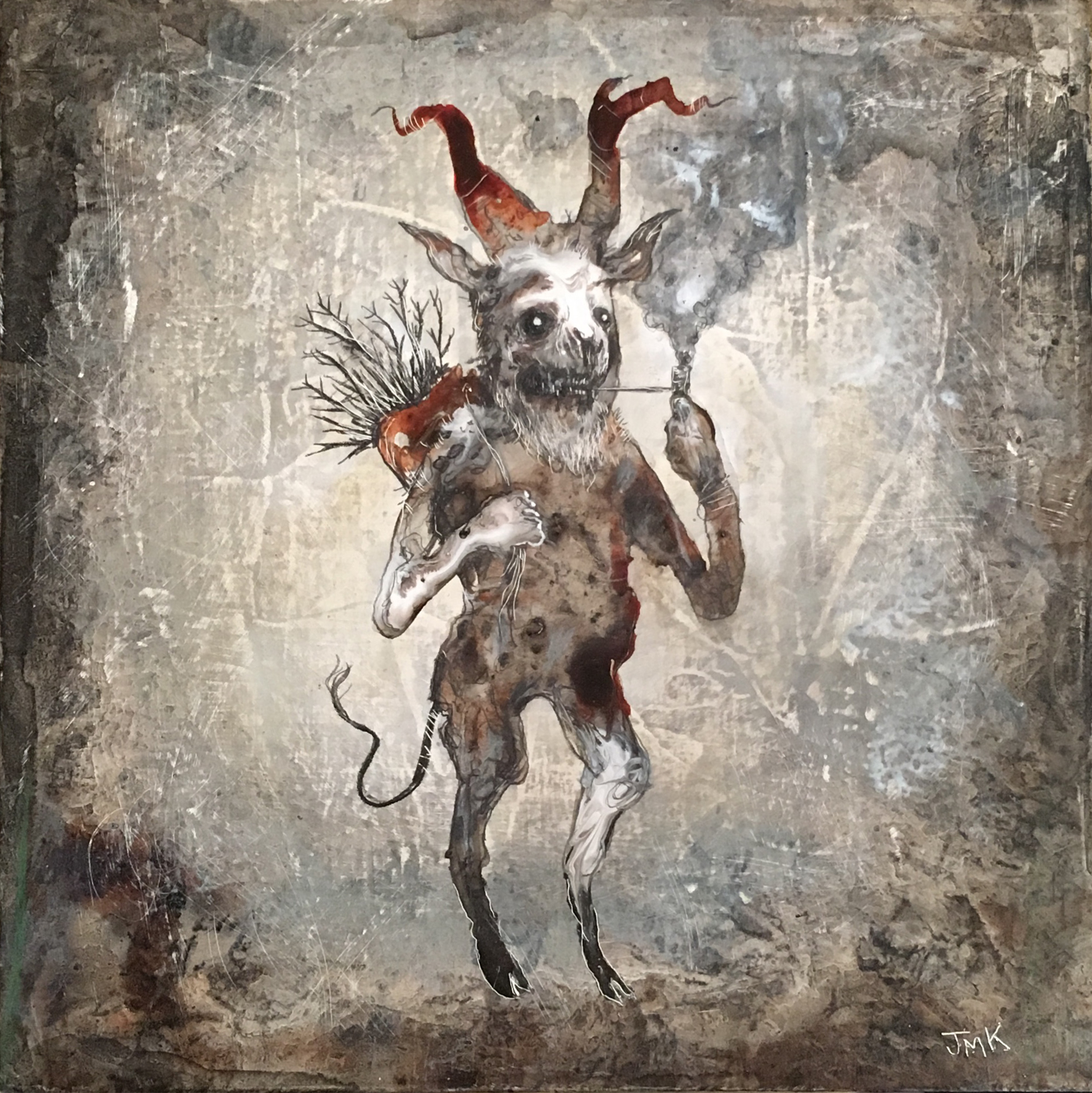This detailed painting vividly captures a hellish and sinister anthropomorphic goat standing upright on its hind legs, which end in uneven hooves. The creature's color palette consists of red and white hues, with its face appearing burnt and blackened in places, evoking a horrific aura. It smokes a pipe from which emerges a plume of smoke that intriguingly forms a human-like face. The goat's face is a disturbing blend, resembling a bunny's nose with sharp teeth and pure white pupils set in black sockets, further enhancing its nightmarish look. Adorned with two horns that transition from light gray to dark red, the head is crowned with an ominous presence. It carries a satchel or backpack brimming with barren, spindly sticks over its back. The background features a dark brown and gray watercolor-esque gradient, adding to the painting's bleak and eerie atmosphere. The overall style is painted and sketchy, contributing to its haunting appearance.